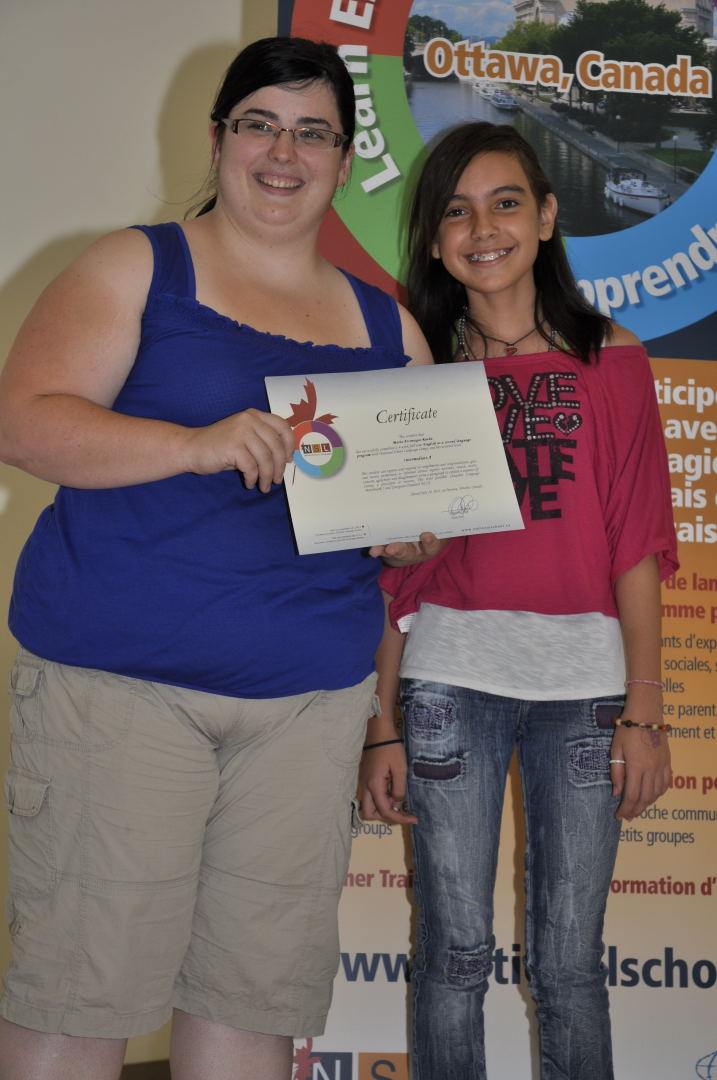In this image, a teenage girl is being presented with a certificate by a woman standing beside her. Behind them, a wall displays a sign that reads "Ottawa, Canada," accompanied by a partially obscured logo and some additional text. The woman, probably in her 30s, has dark hair pulled back and is wearing glasses with copper-colored frames. She is dressed in a blue tank top and khaki cargo shorts, and she is smiling warmly as she holds up the certificate. The teenage girl has black hair and is also smiling. She is wearing a pink top with black lettering that appears to say "Love" or "Love Me, Hate Me," over a gray and white undershirt, paired with stonewashed jeans. The girl has braces and is accessorized with several bracelets on both wrists and a ring on her left thumb. They both appear to be enjoying the moment.